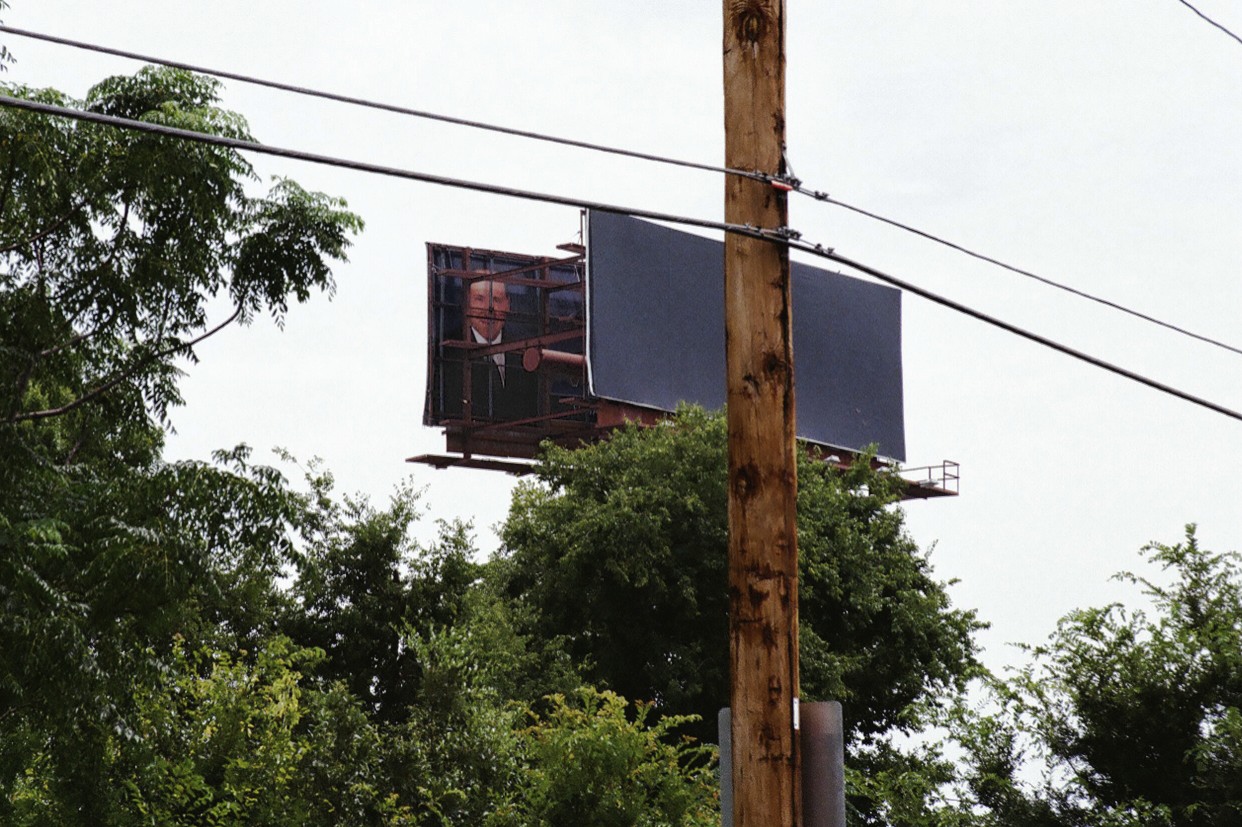In this detailed outdoor image, a serene setting of nature and infrastructure coexists. On the left, a cluster of trees with lush, dark green leaves begins to emerge. Among them, the tallest tree stands prominently at the far left. Dominating the foreground is a brown telephone pole, extending vertically from the bottom edge of the image. Attached to the pole are two gray telephone wires running horizontally. In the background, a square, gray sign is partially visible, behind which the edge of a person's face can be discerned. More foliage appears in the bottom right-hand corner, while the backdrop of the scene is a clear, white sky, enhancing the contrasts within the composition.